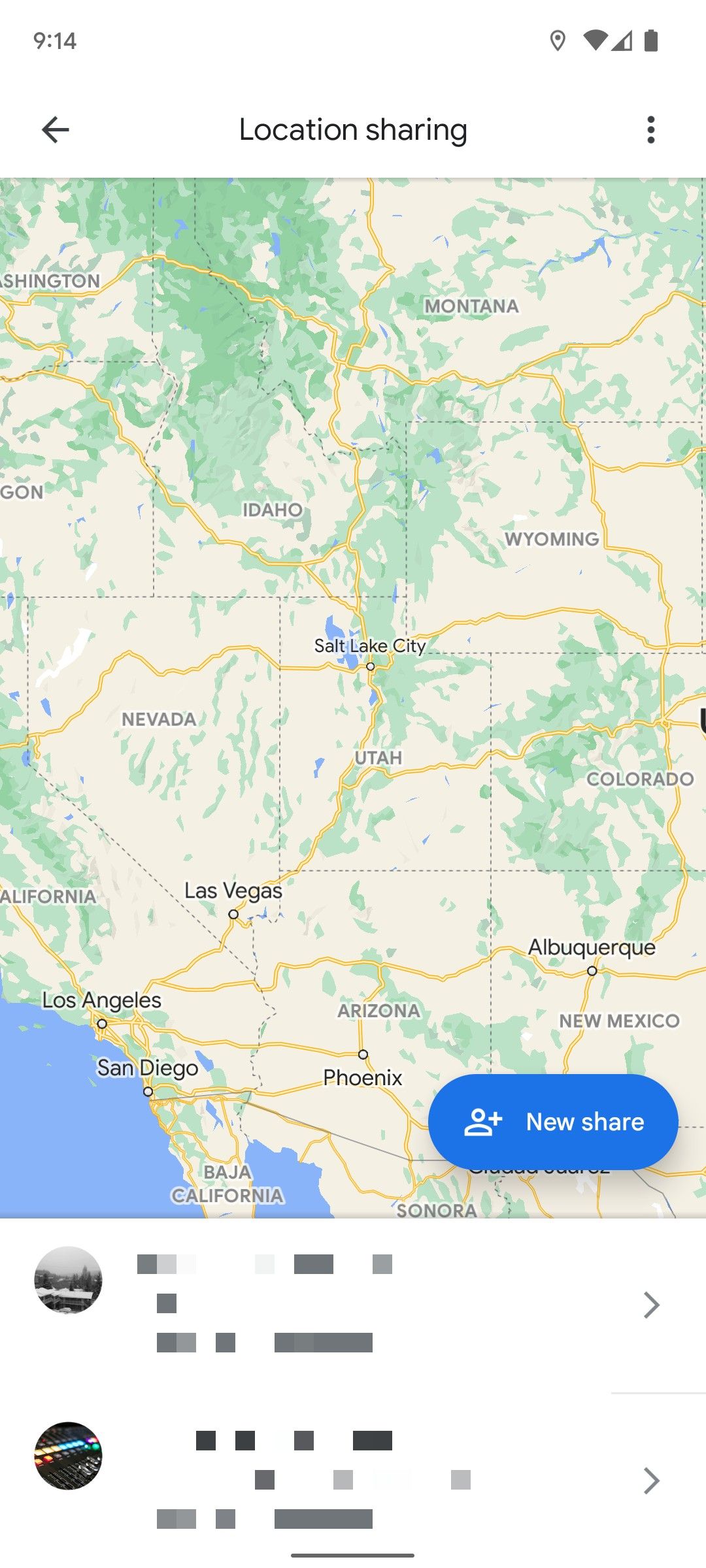Screenshot of a mobile application displaying a map interface focused on the western United States. At the top of the screen, in a white header, "Location Sharing" is prominently displayed. To the left of this text, a back arrow icon is visible, allowing users to return to the previous screen. On the right side of the header, a vertical three dots icon provides access to additional options.

The map itself spans from Montana in the north down to New Mexico in the south, and from California on the west to parts of Utah and Colorado on the east. Notably, only the northern half of California is visible, including cities such as Los Angeles, and similarly, only the southern half of Washington State is displayed. This focal area provides a geographical context for the user's shared location.

In the bottom right corner of the map, a prominent blue, pill-shaped button labeled "New Share" invites users to initiate a new location-sharing session. Below the map, there are two comments that have been censored and blurred out, ensuring that any sensitive information is obscured and unreadable.

This screenshot effectively captures the essential elements of the app interface, emphasizing location sharing features and geographic coverage.